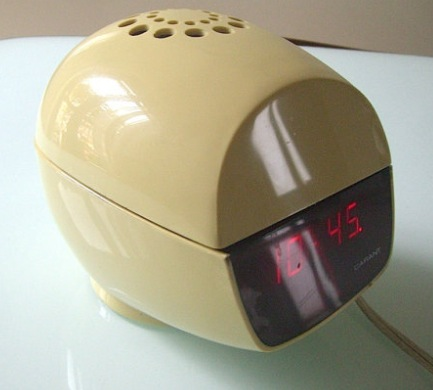A beautifully nostalgic photograph captures a vintage alarm clock resting on a pristine white nightstand. The clock, reminiscent of the 1950s and 60s era with its beige hue and Art Deco design, exudes a timeless charm. The circular, almost egg-shaped clock features a flat front surface and a classic face displaying the time as 10:45 in aged red numerals. The beige color of the clock, whether a result of its original design or the natural yellowing of old plastic, adds to its antique appeal. Small perforations along the top enhance its floral, decorative look. A cord trails from the back of the clock, disappearing out of the frame, hinting at its electric nature.

The nightstand itself is white, possibly made of plastic, glass, or marble, with a sleek, flat surface that subtly reflects the clock, suggesting a glossy finish. Shadows cast by this setup add depth to the image, with one extending towards the back of the nightstand. The background maintains a soft beige tone, complementing the color palette of the clock and enhancing the overall vintage aesthetic. Faint reflections on the clock include glimpses of windows and possibly some plants, adding a hint of life and movement to this still-life composition.